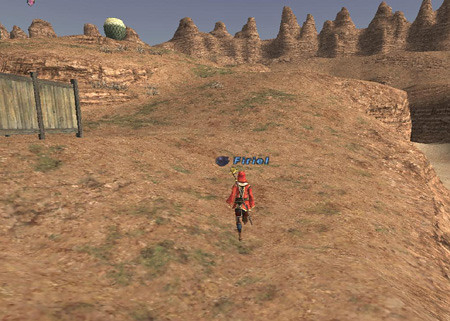This detailed color image appears to be a screenshot from a video game, featuring a character named "Firiel" walking atop sandy dunes in a rugged, rocky terrain. The scene resembles a place similar to the Grand Canyon, with numerous rocky cliffs and peaks visible in the background. The terrain is predominantly reddish-brown with patches of green grass. The sky overhead is a clear, grayish-blue, devoid of clouds. To the far left of the image, there is a wooden fence. The character, Firiel, who has his name displayed above him in blue text, is dressed in a red shirt and black pants. He has a weapon strapped to his back and carries a staff with a satchel. The overall graphics appear to be somewhat dated, with a low poly count, contributing to the scene’s retro video game aesthetic.